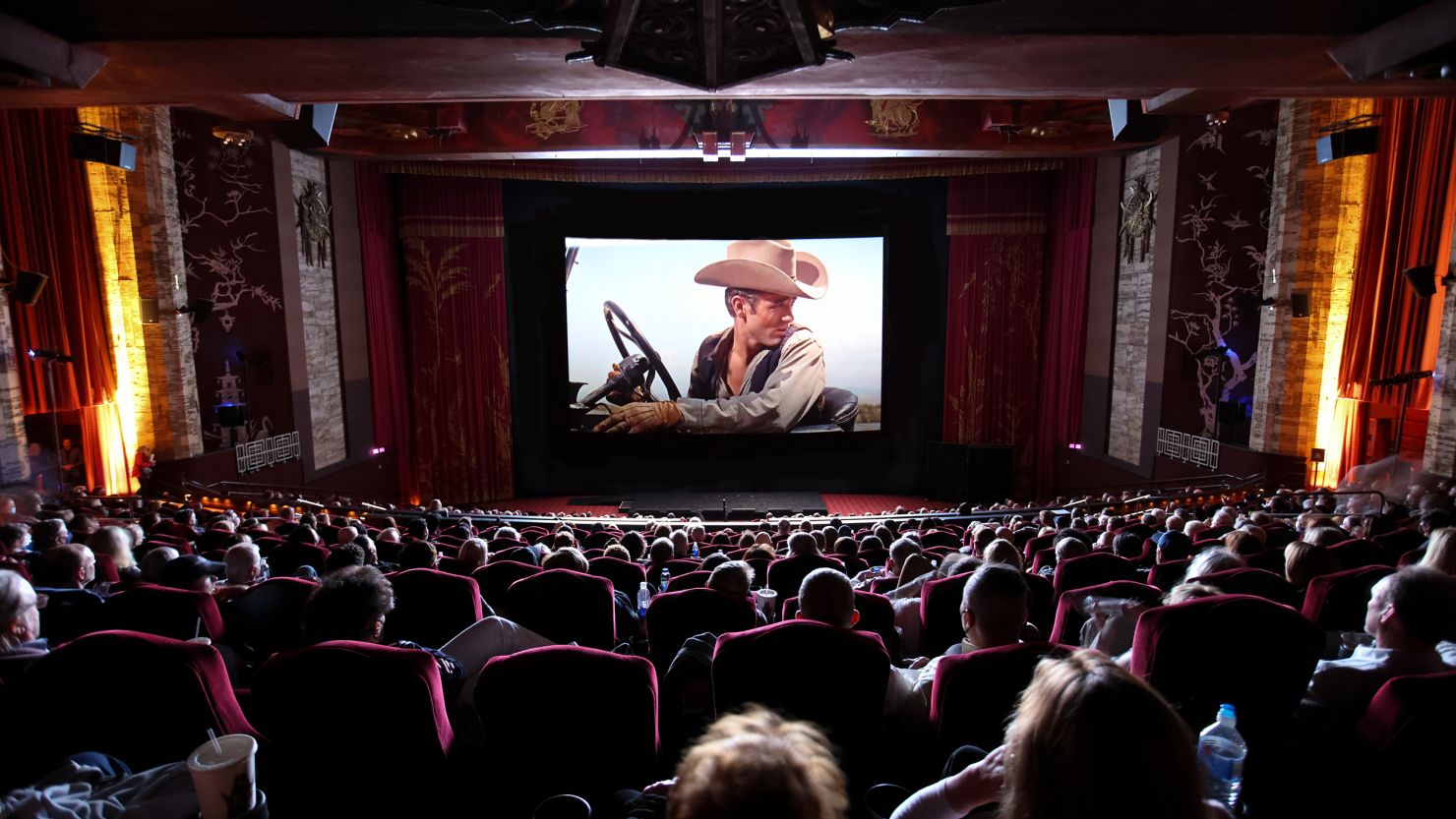The photo captures an opulent, vintage movie theater seen from the back, filled with over a hundred people seated in red velvet seats. The theater's grand design includes intricate gold designs around the screen, elaborate red and gold curtains on either side, and decorative elements on the walls. A movie is playing on the screen, featuring James Dean in a scene from "Giant," where he's wearing a cowboy hat and a brown vest, sitting in a convertible car, and looking over his left shoulder with a concerned expression. The scene is accented by his white long-sleeve shirt and brown gloves, with the open car revealing the daytime backdrop. The dimly lit theater's lavish interior, combined with the classic film scene, evokes a rich, nostalgic ambiance.